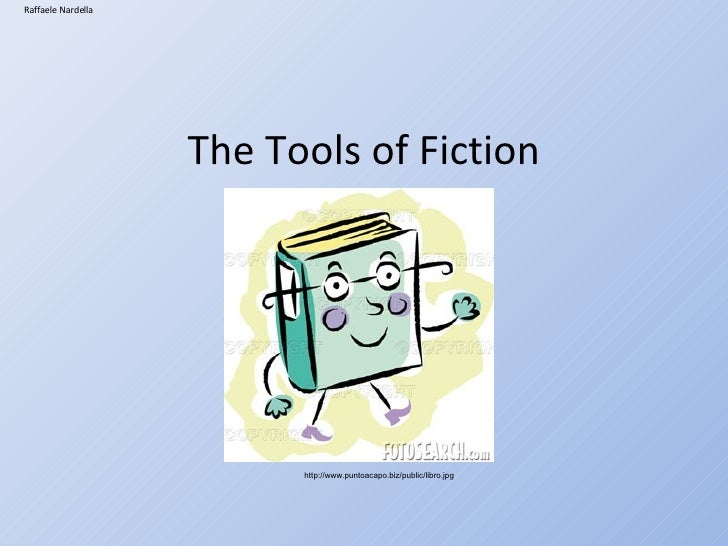The image appears to be an illustration, likely from a book, article, or website page, featuring a sky-blue background with the title "The Tools of Fiction" prominently displayed in black print at the top. Below the title, there is an anthropomorphized book that resembles a person, adding a cartoon-like feel to the image. The book has a light sage green color with a darker green spine. It is depicted as having a face, complete with glasses, eyes, a funny nose, and a smile made from simple lines. Adding a touch of whimsy, the book character has rosy, purple cheeks. The book features skinny arms and legs, with green hands and purple shoes, suggesting movement as its arms and legs are positioned to imply it is walking. The character is surrounded by a fluffy, yellowish cloud. Additional details include a small text in the top left corner that reads "Rafael Nardella" and the bottom text stating "Photosearch.com" with the URL "http://www.puntoacapo.biz." The overall color scheme consists of light blue, sage green, turquoise, yellow, purple, black, and white, lending a vibrant and engaging aesthetic to the image.